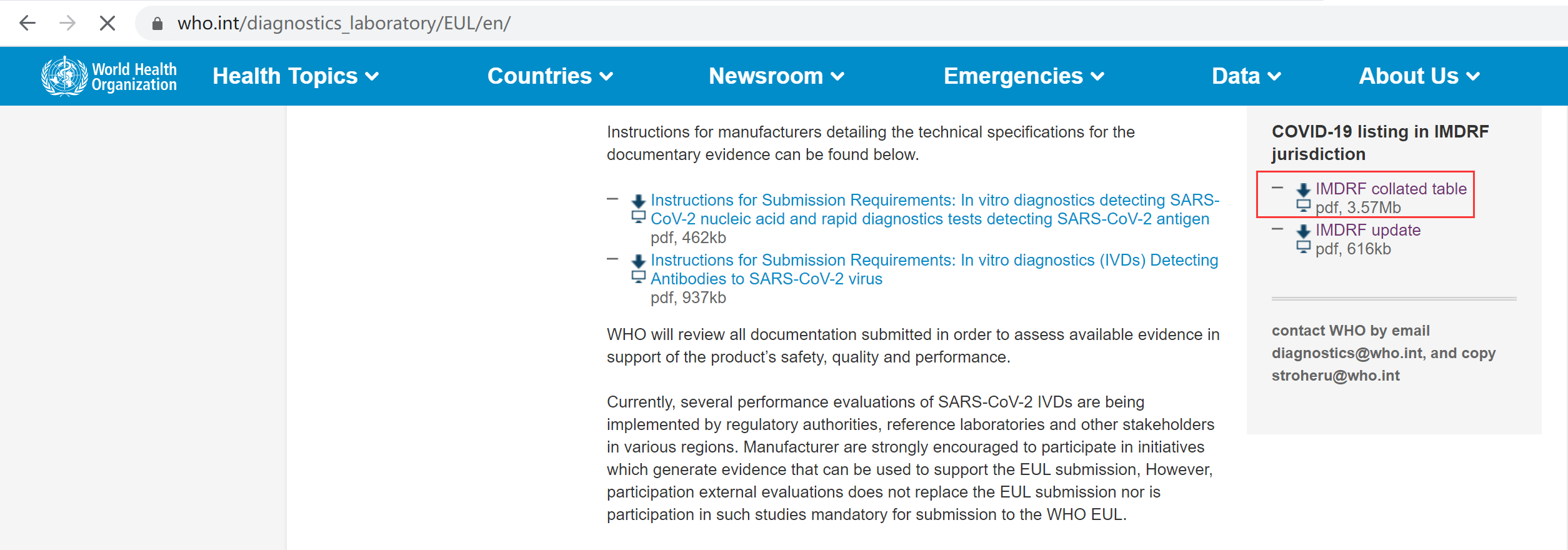The image displays a webpage from the World Health Organization (WHO). At the top of the page, there is a prominent blue banner stretching across the width of the website. The overall theme of the page revolves around health-related information. The layout incorporates a variety of colors, with black text set against a white background, and some blue lettering in the middle of the page.

On the right side, there is a section dedicated to COVID-19, titled "COVID-19, list of IMDRF jurisdictions." A red square highlights this section, stating "Highlighting IMDRF collated table," followed by a file size of 3.57 megabytes. Below this, a similar entry is listed, but it indicates a file size of 616 kilobytes.

At the top of the webpage interface, navigation icons are visible, including a back arrow, a forward arrow (which is slightly faded), an X, and a lock symbol. The webpage URL displayed is "who.int diagnostics laboratory, E-U-L-E-N." 

This detailed description captures the key elements and visual layout of the WHO webpage focused on COVID-19 and IMDRF jurisdictional information.